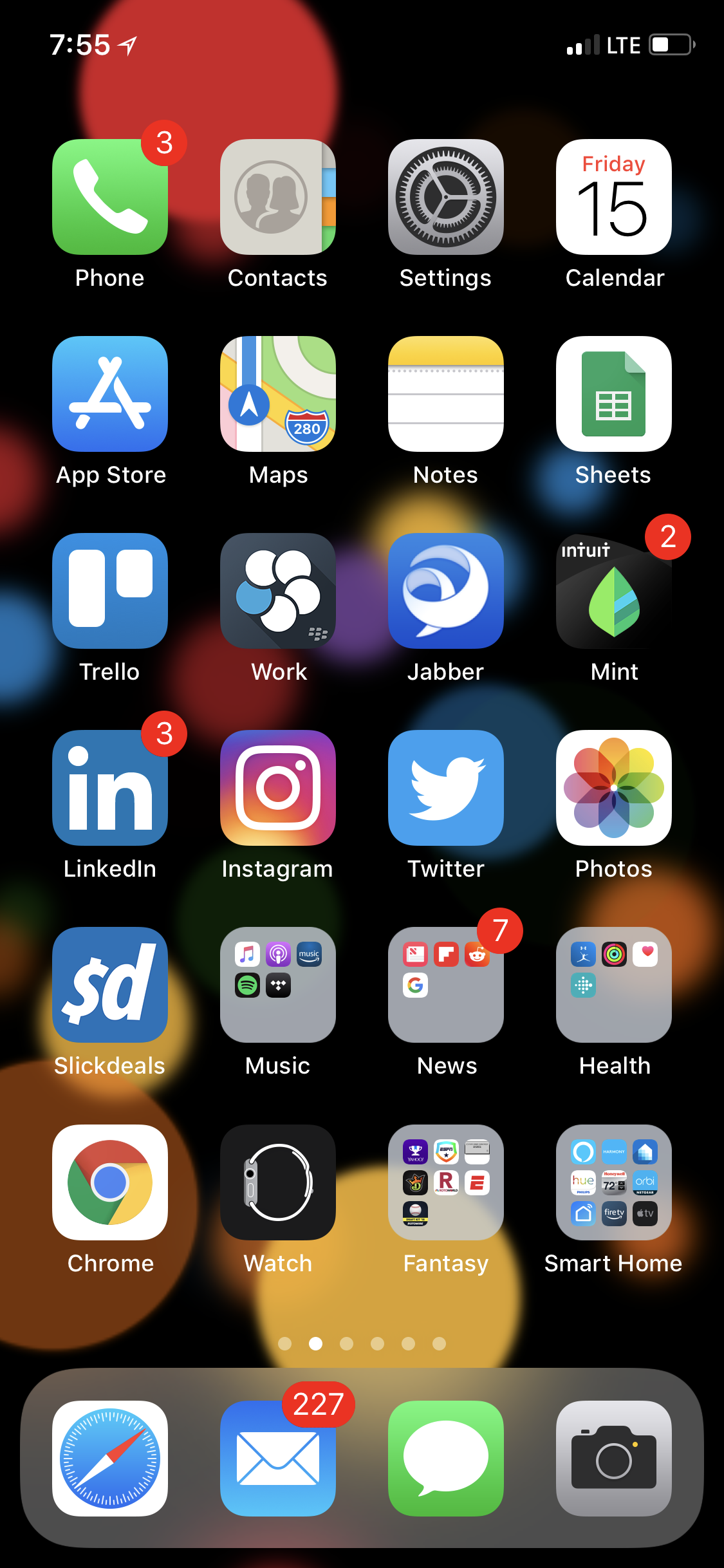Screenshot of a smartphone home screen captured at 7:55 am, indicated by the time displayed at the top left corner. On the top right, there are cellular signal bars with two bars present, and the letters "LTE" indicating the network connection.

The home screen displays a series of app icons arranged in a grid format:

- First row: Contacts and Settings.
- The date is listed just below them, stating "Friday the 15th."

Followed by additional app tiles:

- Second row: App Store, Maps, Notes, and Sheets.
- Third row: Trello, Work, Jabber, and Mint, with a notification badge showing "2" on Mint.
- Fourth row: LinkedIn with a notification badge showing "3", Instagram, Twitter, and Photos.
- Fifth row: Slick Ideas, Slick Deals, Music, and News with a notification badge showing "7".
- Sixth row: Health, Chrome, Watch, Fantasy, and Smart Home.

At the very bottom of the screen, there are four more icons:

- Compass
- Email with a significant notification count of "227"
- Messages (Bubble icon)
- Camera

Each icon represents the user's mix of productivity, social, utility, and communication apps.